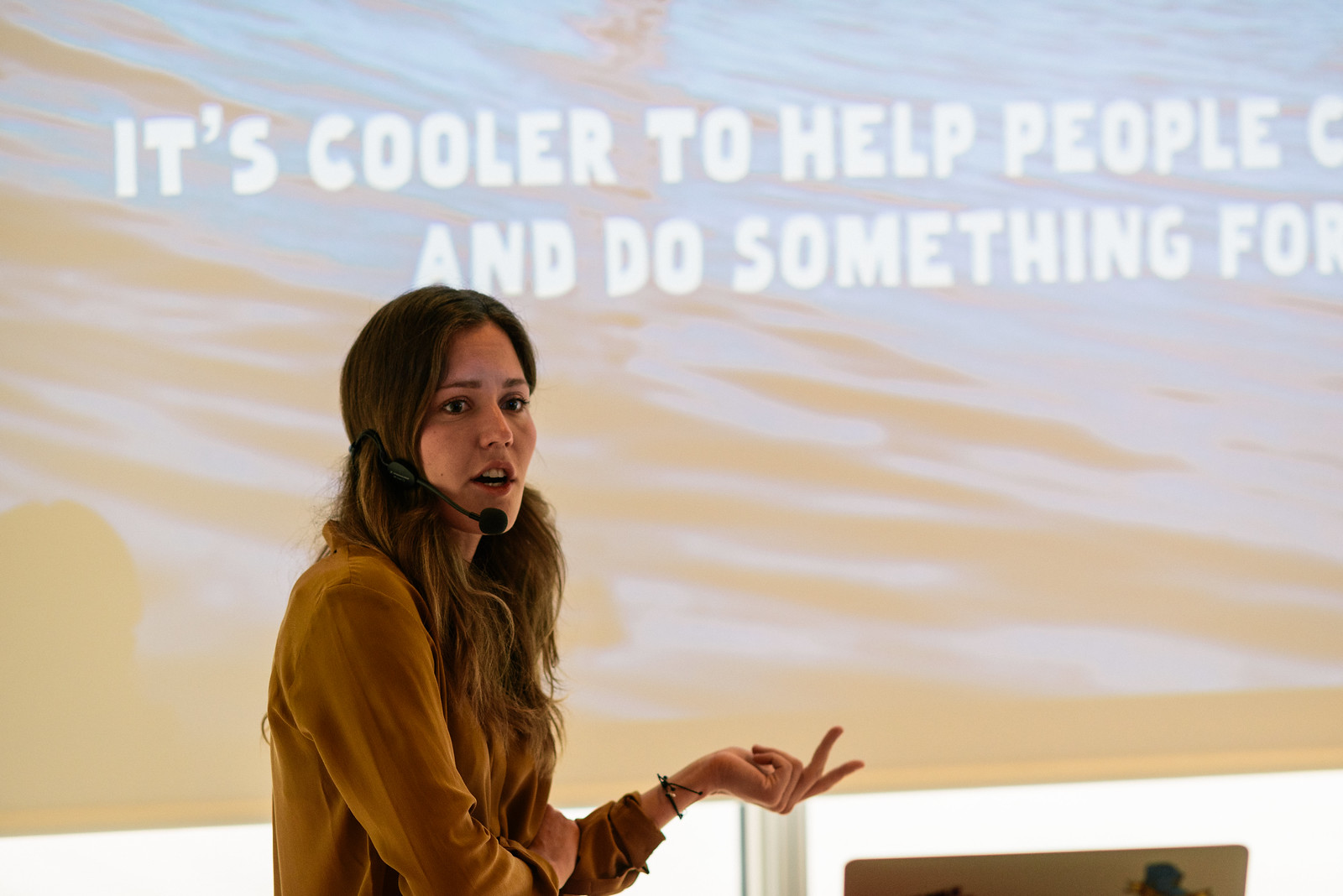The landscape-oriented color photograph depicts a woman in her early thirties standing slightly left of center, addressing an unseen audience. With long dark hair and a headset microphone under her chin, she gestures animatedly with her left hand as she speaks. The woman, dressed in a gold or brown long-sleeve sweater, gazes out towards the viewers with an attentive expression. The setting is indoors, likely midday, as suggested by the lighting.

Behind her, a projection screen on a silver post displays an image of water with partially visible white block text. The readable portions of the text state, "it's cooler to help people," and, "and do something for," before being cut off. Below the screen, a portion of a white wall and the top of an open laptop are visible. The scene projects an atmosphere of a formal presentation or seminar, as indicated by the woman's poised stance and the professional setting. The colors in the image, consisting of white, tan, brown, black, blue, and gray, complement the overall compositional elements, enhancing the detailed realism of the photograph.